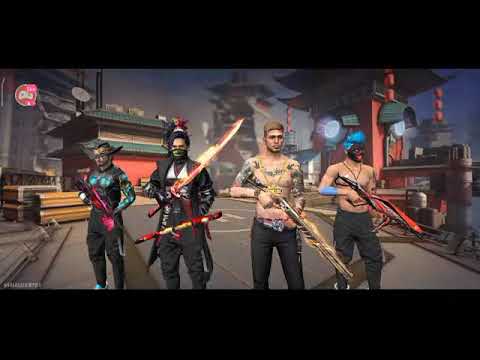The image is a highly detailed screenshot from a video game displaying four distinct characters in a visually striking and futuristic urban environment. All four men are standing side by side on a street or possibly a rooftop with a helipad, surrounded by buildings reflective of East Asian architecture complete with curved roofs and tile details. The two characters on the left are clad in black bodysuits; one has patches of blue on his chest and arms, while the other dons a samurai-like outfit with a face mask reminiscent of modern tactical gear and is equipped with laser swords. The two characters on the right are shirtless with black pants; one sports tattoos covering his chest and arms along with a golden chain, and the other wears a blue helmet with his face painted black and a full face mask. Both are armed with guns. The background includes a variety of buildings, ranging from a tall distant tower to shorter red and brown structures, adding to the rich, cyberpunk-inspired setting.